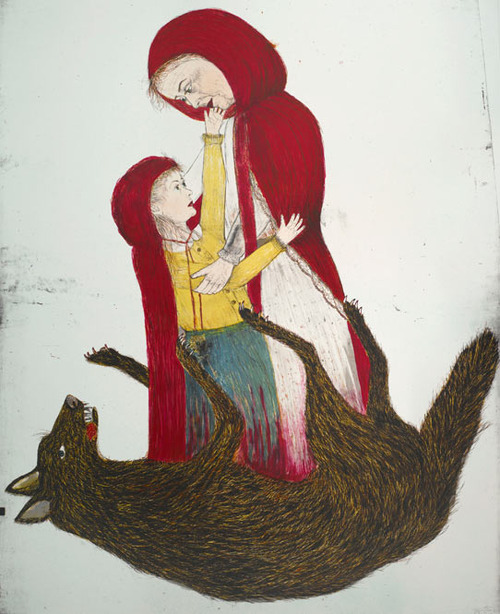This vertically aligned, rectangular piece of artwork, likely done on paper, presents a detailed, hand-drawn or painted scene with a predominantly light gray to off-white background, accented by various smudges of color. At the center, a woman and a little girl, both wearing red hooded capes, occupy the focal point. The woman stands facing left, adorned in a red cape over a white gown, gazing downwards at the child. The little girl, positioned in front of the woman, mirrors her red hood and cape, complemented by a long-sleeved yellow blouse and either a pink skirt or blue bottoms. Her arm reaches up to touch the woman's face, while the other rests around the woman's waist.

Below them lies a dead wolf, its body rendered in dark to medium brown hues, with its legs seemingly entangled around the two figures. The wolf is depicted upside down, eyes and mouth open, revealing sharp teeth and a protruding tongue. Red streaks emanate from its stomach, suggesting blood, and a similar spot of red is visible near its mouth.

The composition includes an array of colors—red, yellow, blue, pink, purple, and various shades of brown—against the largely empty, smudged background, giving the artwork a haunting ambiance reminiscent of a dark fairy tale.